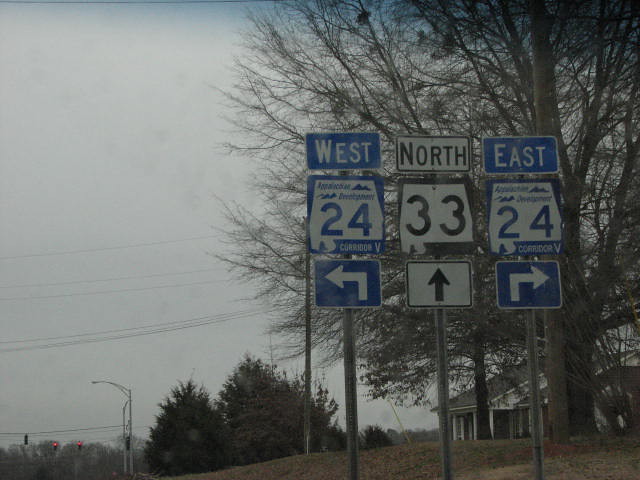In this image, taken from an eye-level perspective slightly looking up, three street signs prominently stand against the backdrop of a vibrant neighborhood. The signs, mounted on a steel rod slightly right of center, extend to about the middle of the frame. 

At the top of the left side, a sign with a white rectangle bears the word "West" alongside a blue square labeled with a bold number "24." Below this, a smaller white square features an upward arrow pointing left. Adjacent to it is a vertical sequence of signs; the top sign reads "North" in black lettering on a white background, followed by another square with the number "33." Concluding this row, a white sign with a black arrow points straight ahead. On the far right, a blue rectangle is marked with "East," with a subsequent blue-bordered white square showing the number "24." Below this, a blue square displays an upward arrow pointing right.

Behind the signs, a large tree and partial view of a white house with a gray roof are visible. The house sits almost to the bottom edge of the image, accompanied by a glimpse of its green lawn. To the left, two sizable trees and a streetlight rise above, leading the eye towards two red traffic lights in the lower left corner amid distant trees. The scene is crowned with a dark blue sky that peeks through the foliage, adding depth and contrast to the setting, which appears to be a somewhat residential area. The colors in the image span from the gray of steel to the vibrant blue and white of the signs, with touches of red, green, and the underlying tones of the natural and built surroundings.